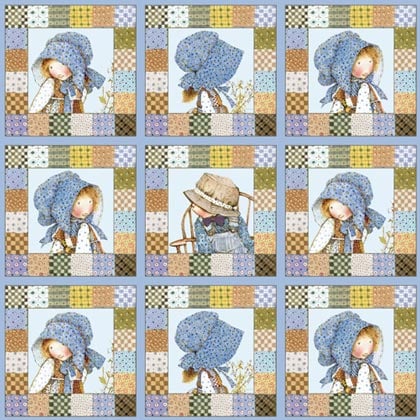This is an illustration mimicking a quilt, featuring a three-by-three grid of square panels depicting a doll-like young girl and one boy, styled in a Holly Hobbie fashion. The central image showcases a young boy in overalls, a blue T-shirt, and a beige bucket hat, looking to the left with his face partially obscured. Surrounding him are eight panels of the girl, each accentuated by her iconic oversized blue bonnet. She poses differently in each frame: facing left, right, downward, and in profile. The images depict her head and upper body in muted colors, primarily neutrals, browns, blues, and yellows. Each panel is surrounded by patchwork designs of abstract checkered fabric in varied colors like yellow, green, white, purple, and orange, separated by a thin blue ribbon, which also borders the entire illustration.